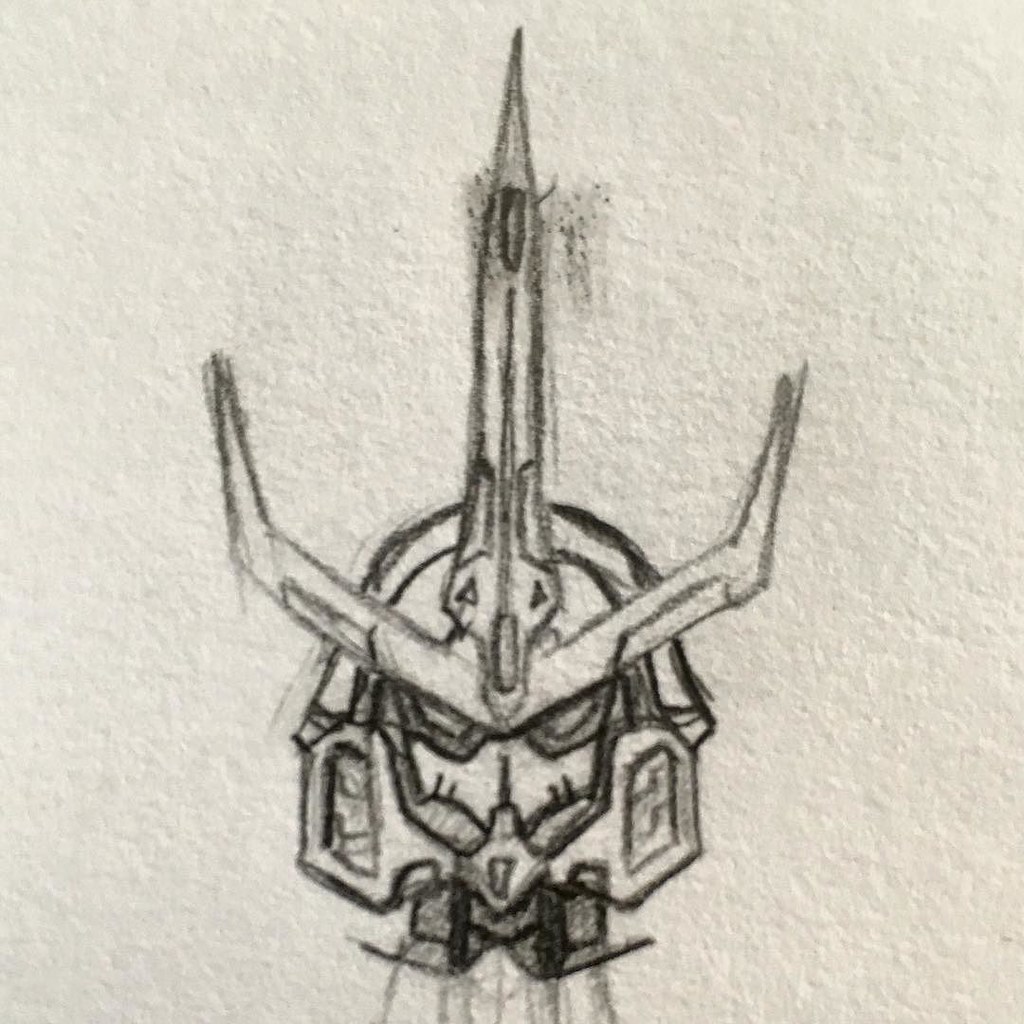This detailed black-and-white sketch, likely created with pencil on a textured surface resembling a painted wall, portrays a fantastical, sci-fi creature with an intricate design. The central figure features a long, narrow head with triangular eyes that might suggest an alien appearance, complete with a couple of eyelashes on each eye and a mask-like structure over its face. The creature wears an elaborate headdress that includes elements reminiscent of horns or arms, giving an impression of a deer head piece or possibly even organic appendages. The headdress also incorporates a striking sword-like adornment extending vertically from the top, with the hilt resembling bird wings folded upwards. Additional features include a helmet-like structure that covers the head down to the base of the neck, emphasizing a hardened, possibly warrior-like, insectoid visage with goggles and a pronounced, ant-like jaw. The smudged and roughly textured background adds a sense of depth and unease, while finer, sketchy lines at the bottom suggest a partially rendered neck or extension of the figure. The overall composition is detailed and direct, with the figure facing forward, engaging the viewer with its complex and enigmatic appearance.